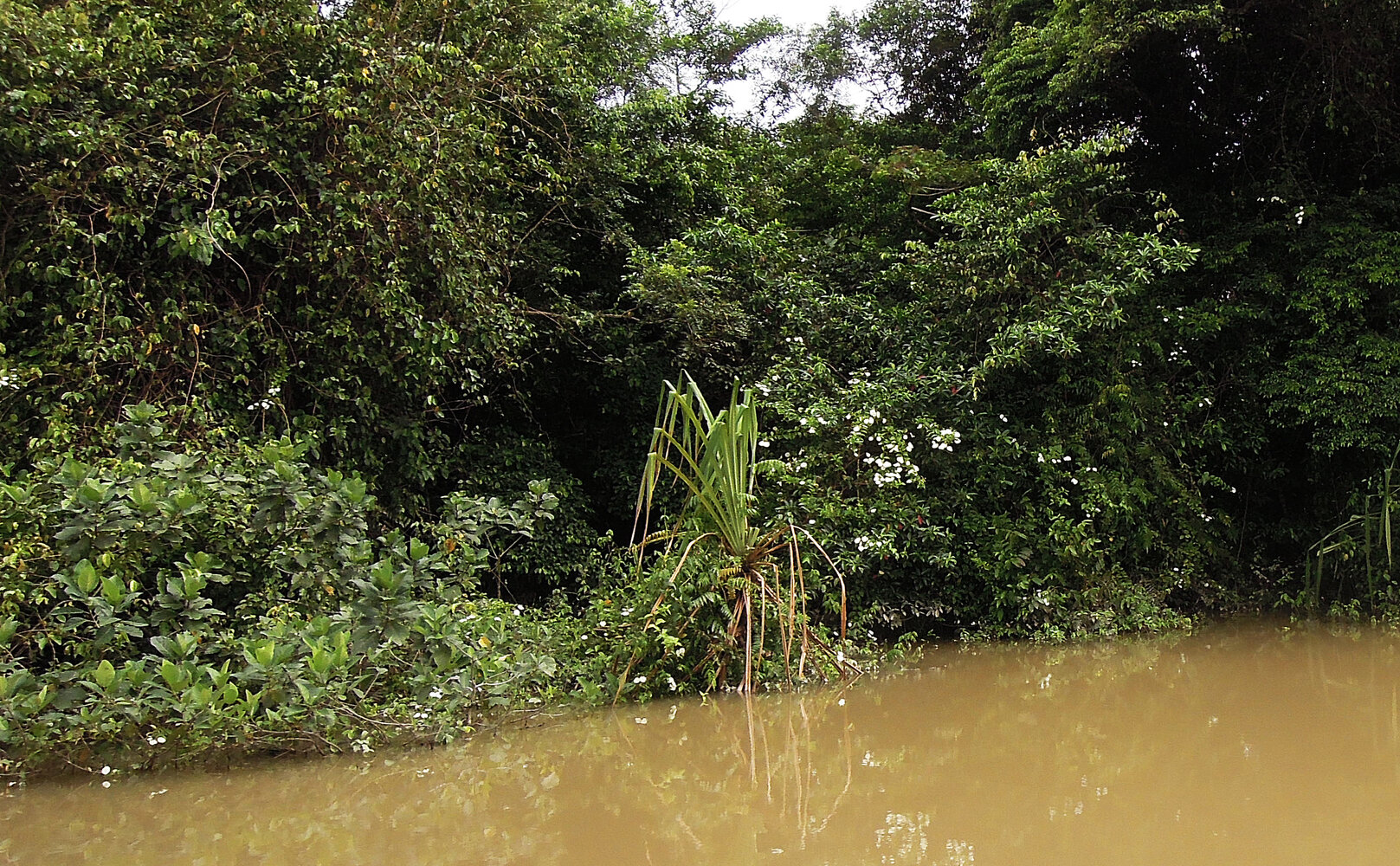This detailed image depicts a tranquil swamp-like landscape bathed in sunlight, with a dominant, extremely muddy pond or body of water occupying the lower portion of the frame, notably more to the right side. The murky water presents a brownish-green hue, reflecting the rich greenery of the overhanging trees and vegetation that give the scene a lush, vibrant atmosphere. The dense array of dark green trees and diverse plants, including some growing directly out of the water, forms a thick, almost impenetrable backdrop. Among the greenery, a flowering bush displays small white blossoms, adding a touch of contrast. In the center of this verdant setting stands a distinctive plant with long, slim, bending leaves that are lighter green tipped with red and brown. The top center of the image just barely shows a glimpse of white sky, suggesting a sunny day and emphasizing the dense, swampy environment below.